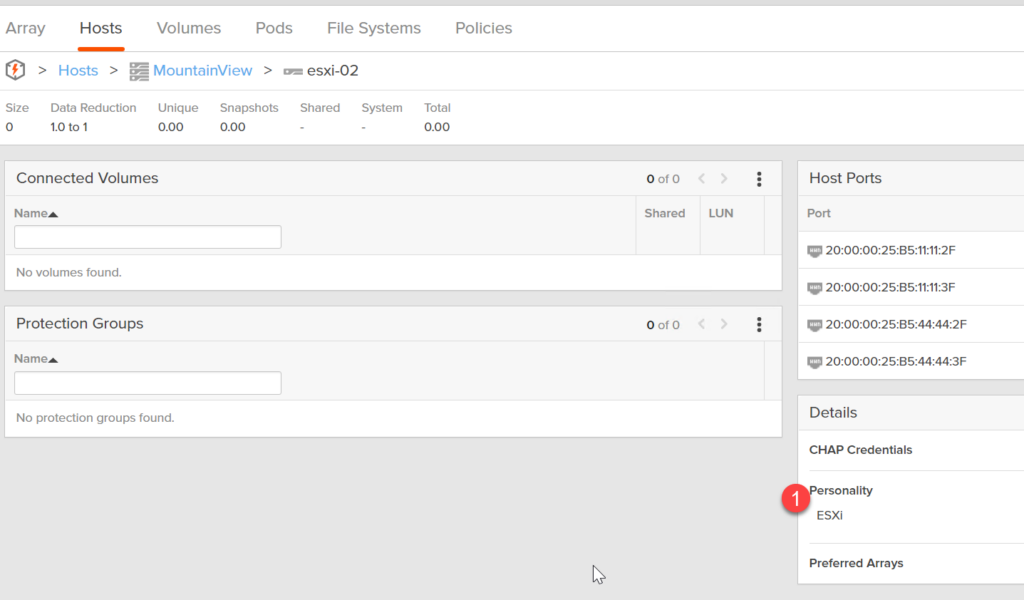This image captures a screenshot of a webpage displayed on a computer screen. At the top of the page, a navigation bar lists several categories: "Array," "Host," "Volumes," "Pods," "File Systems," and "Policies." Below this, in the subsequent section, there is a highlighted block featuring a red squiggle. The block contains the blue-labeled terms "Host" and "Mountain View," followed by "ESXI-02."

Further details in the section include:
- Size: 0
- Data Reduction: 0
- Unique: 0
- Snapshots: 0 (intended to be displayed as 0.00)

Beneath this block, there is a "Connected Volumes" section. The "Name" field is empty, indicating no name has been provided. Adjacent to it, under "Protection Groups," there is an ascending triangle icon next to the message "No protection groups found."

To the right, an area labeled "Host Ports" contains four clickable icons. Additional fields include "Details," "CHAP Credentials," and "Personality," with the label "ESXI" highlighted. Notably, this section features a red circle with the number "1" in white, which stands out. Finally, there is a mention of "Preferred Arrays."

The overall layout appears to be part of a user interface related to server or storage management, with various details about host configuration and data management tools prominently displayed.